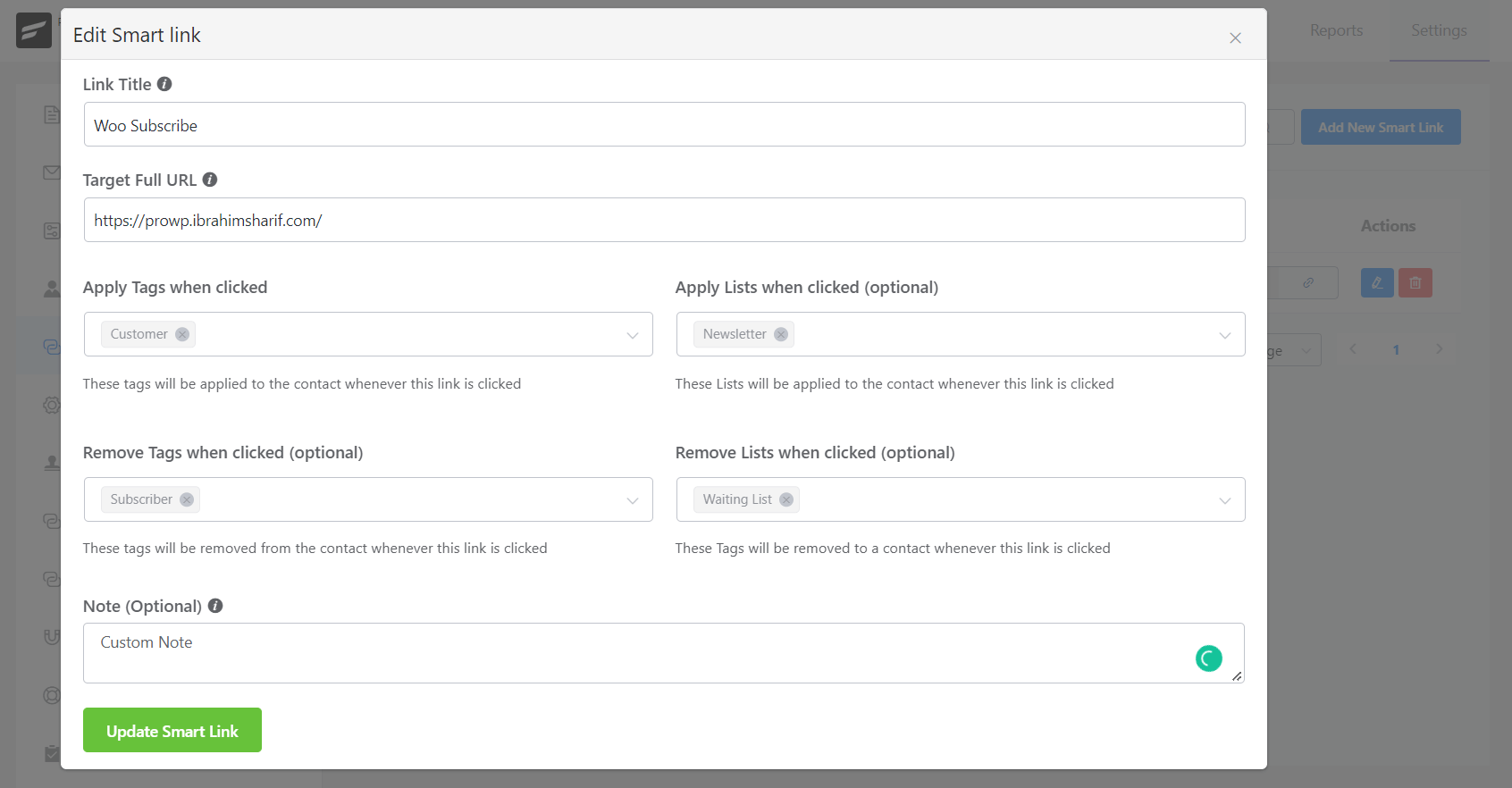The image displays a user interface for editing a smart link, set against a white and grey color palette. The background is entirely white, providing a clean and minimalistic look. The interface features a total of seven fields, each designated for specific details about the smart link. 

The fields are arranged as follows:

1. **Link Title**: This is the first field and is meant for entering the title of the link.
2. **Target Full URL**: The second field, used for inputting the full URL that the link targets.
3. **Apply Tags When Clicked**: The third field, along with the fourth field, is arranged horizontally.
4. **Apply List When Clicked (Optional)**: Placed next to the third field, this is optional.
5. **Remove Tags When Clicked (Optional)**: The fifth field, positioned horizontally alongside the sixth field.
6. **Remove List When Clicked (Optional)**: The sixth field, also optional.
7. **Notes (Optional)**: This final field spans the entire width of the interface, with no other field next to it.

At the very top of the interface is the title “Edit Smart Link.” The action button "Update Smart Link" is prominently highlighted in a green rectangle at the bottom of the interface. The text on the button is written in white, ensuring high visibility and ease of interaction.